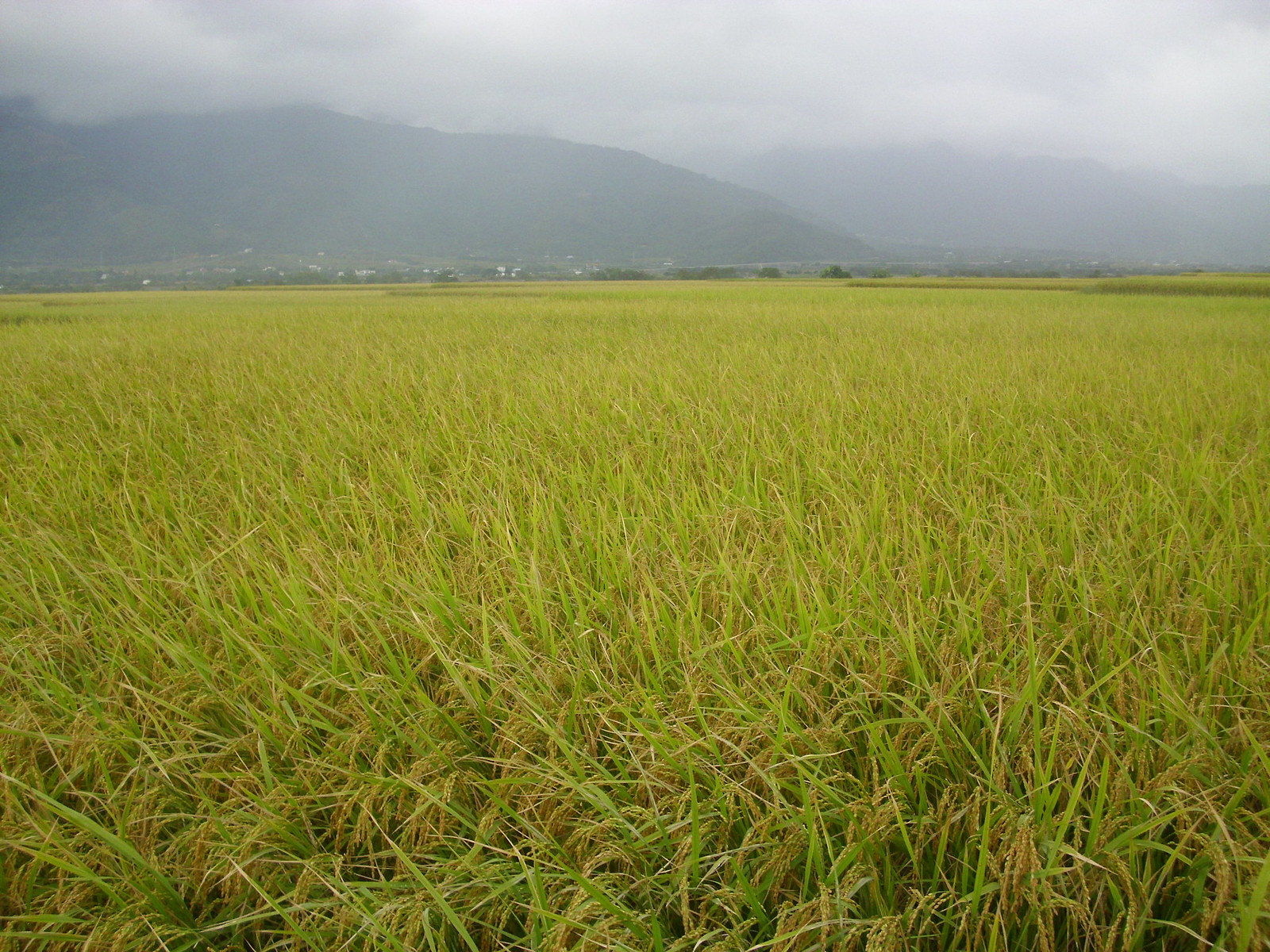The image depicts a large, square close-up of a tall grass field that extends from the bottom up to about two-thirds of the frame. The blades of grass in the foreground show a mixture of green and light brown hues, with some of the taller blades curving over at the top. The middle section of the image is dominated by the field of grass, punctuated with scattered brown tips, possibly indicating varying stages of growth or different types of crops.

In the background, stretching from the left side to the center, stands the outline of a large hill or mountain. The peak of this landform blends into a sky that is bright but predominantly gray, filled with white and grey clouds. At the base of the hill, one can discern what appear to be houses, buildings, or small villages, mingling with patches of trees and bushes that stretch horizontally across the landscape. This distant scenery, shrouded in the dullness of the cloudy sky, contrasts with the vibrant, varied grasses in the foreground, creating a detailed and serene outdoor setting.